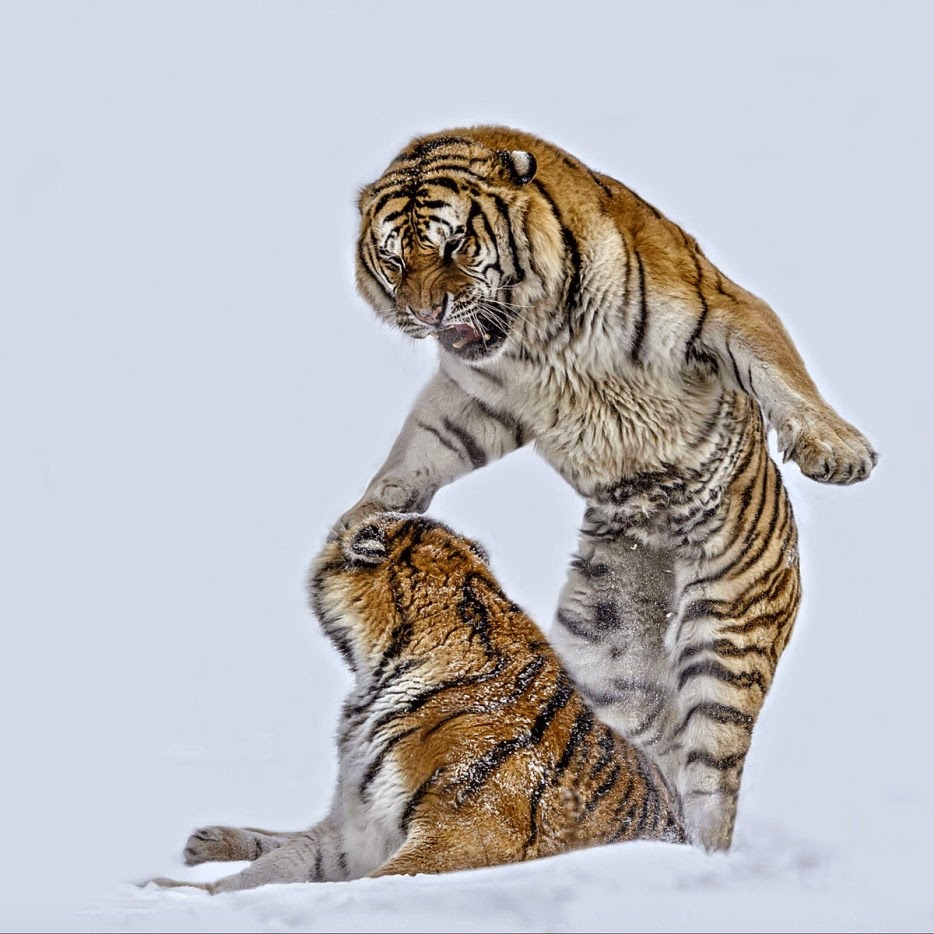In a horizontally aligned photograph, we see two tigers engaged in a fierce battle amidst a snowy landscape. The entire background is dominated by a blanket of white snow, which accentuates the dramatic scene. The tiger on the right stands upright, its body partially turned towards the viewer. This tiger exhibits an angry expression, baring its teeth with a ferocious open mouth, ready to strike. Its powerful right paw is raised, about to land a blow on the face of the second tiger, which lies on the snow-covered ground. The fallen tiger is positioned with its back facing the viewer, its head turned back to look up at its aggressor, covered in snow. Both tigers display the characteristic vibrant orange fur with black stripes on their upper bodies, contrasted by the white of their stomachs and lower legs. The scene, reminiscent of a high-stakes nature documentary, captures the raw intensity and majestic beauty of these powerful creatures in winter.